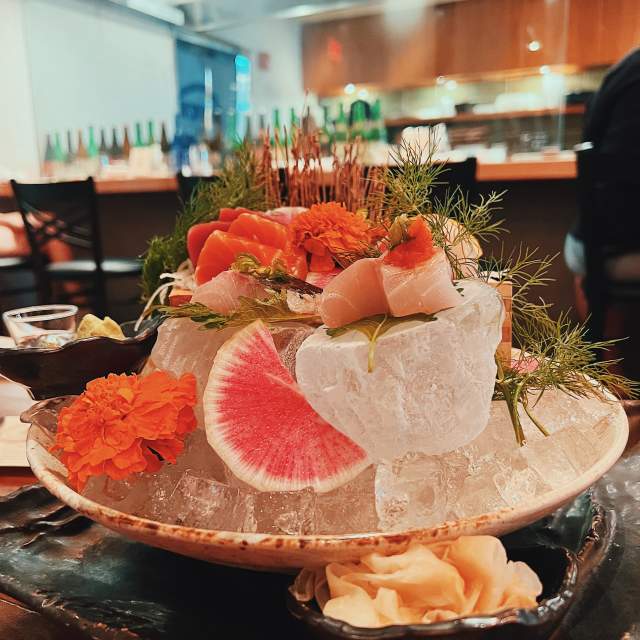The photo captures a highly decorative dish presented on a dark table, possibly in a restaurant or bar setting. Central to the image is a large plate covered in ice chunks, adorned with sprigs of green plants and a pink flower with white tinges. The focal point is a close-up of what appears to be rolled fish, possibly sushi made of salmon or tuna, nestled atop the ice. At the front, a bowl—potentially containing ginger—adds another layer to the presentation. In the background, there's a bar area filled with bottles of alcohol and cabinetry, with an individual seated at the bar on the right-hand side. The scene is rich in colors, primarily reddish pink, light pink, peach, and brown, creating an inviting indoor ambiance.